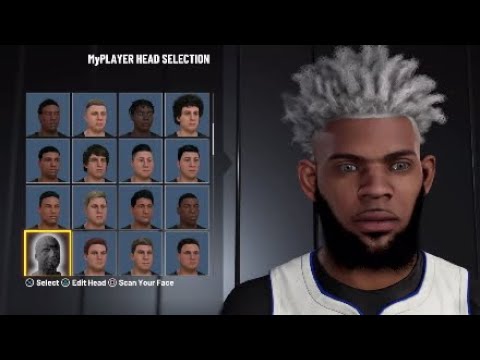The image is a cropped screenshot from the MyPlayer customization section in the NBA 2K video game franchise. At the top left corner, it displays the text "MyPlayer Head Selection." Beneath this title, a large square grid is prominently shown, featuring a selection of 16 different heads arranged in four rows of four. These heads showcase a variety of skin tones and hairstyles. The first head in the third row is highlighted with a yellow box and appears grayed out.

Adjacent to the selected head, a larger image of the face is displayed on the right side of the screen. Below the grid of heads, there are options labeled "Select," "Edit Head," and "Scan Your Face," each accompanied by corresponding controller button prompts for easy navigation. 

The top and bottom edges of the screenshot are bordered by blank, black bars. The background of the scene is reminiscent of a locker room, with gray walls accented by vertical black stripes, adding an authentic sports environment feeling to the customization interface.